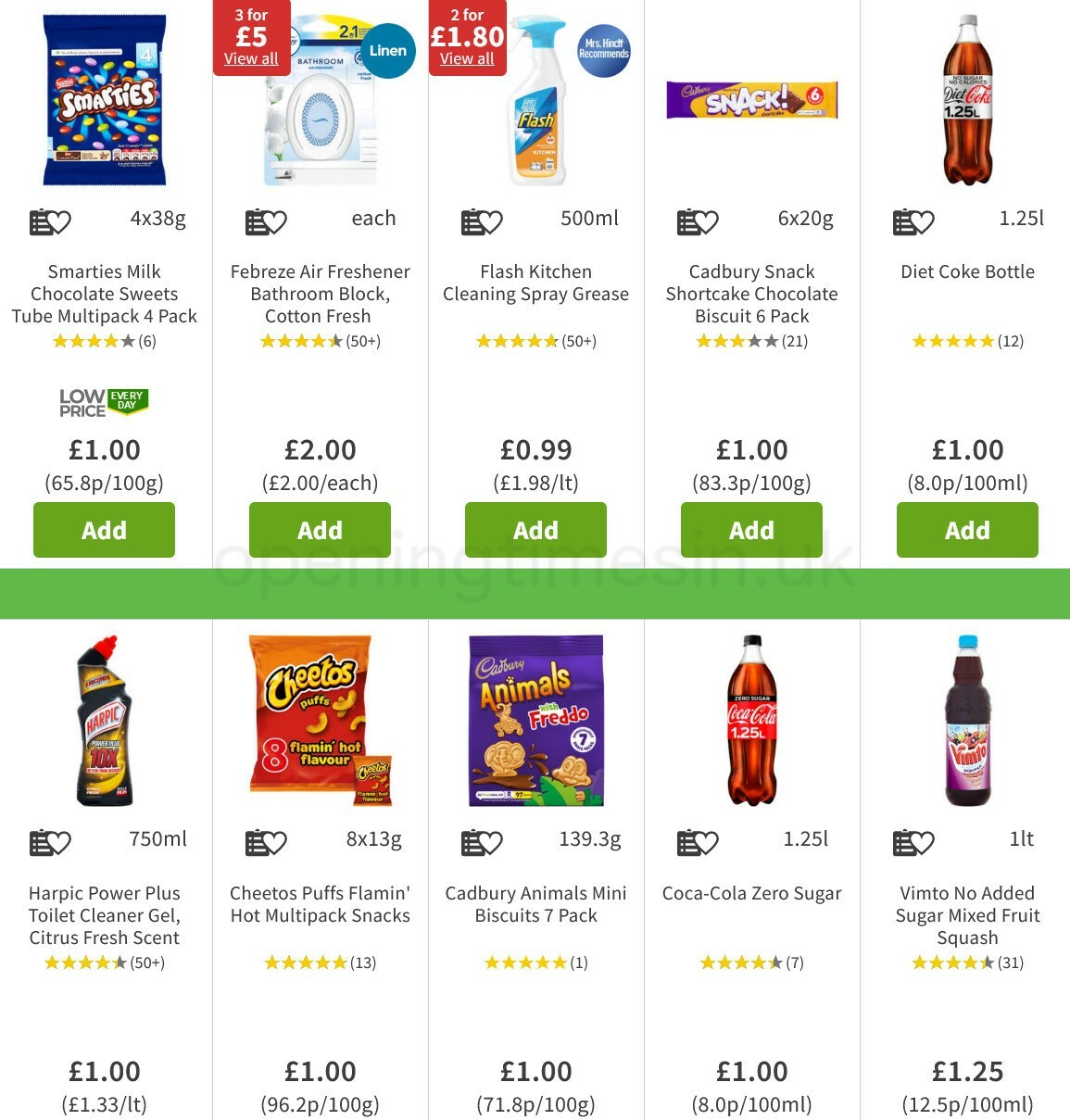The image depicts a web page displaying two rows of product listings, each row containing five products. Each product listing includes an image, details about the product, and purchasing options.

1. **Smarties Candies**:
   - **Image**: A bag of Smarties candies.
   - **Label**: 4x38G.
   - **Title**: Smarties Milk Chocolate Bleach Tube Multi-Pack, Four-Pack.
   - **Rating**: 4 out of 5 stars (6 reviews).
   - **Pricing**: 1 euro, 65.8P per 100G.
   - **Button**: Green "Add" button.

2. **Febreze Air Freshener**:
   - **Image**: Febreze air freshener for bathrooms.
   - **Label**: Each.
   - **Title**: Febreze Air Freshener Bathroom Block Cotton Fresh.
   - **Rating**: 4.5 out of 5 stars (50+ reviews).
   - **Pricing**: 2 euros, 2 euros each.
   - **Promotion**: Red box with "3 for 5 euros View All."
   - **Button**: Green "Add" button.

3. **Flash Kitchen Cleaning Spray**:
   - **Image**: Flash kitchen cleaning spray.
   - **Label**: Each.
   - **Title**: Flash Kitchen Cleaning Spray, Grease.
   - **Rating**: 4.85 out of 5 stars (50+ reviews).
   - **Pricing**: 0.99 euros, 1.98 euros per liter.
   - **Promotion**: Red box with "2 for 1.80 euros View All."
   - **Button**: Green "Add" button.

4. **Cadbury Snack Shortcake Chocolate Biscuit 6-Pack**:
   - **Image**: Cadbury Snack Shortcake Chocolate Biscuit.
   - **Label**: 6x20G.
   - **Title**: Cadbury Snack Shortcake Chocolate Biscuit, Six-Pack.
   - **Rating**: 3 out of 5 stars (21 reviews).
   - **Pricing**: 1 euro, 83.3P per 100G.
   - **Button**: Green "Add" button.

5. **Diet Coke Bottle**:
   - **Image**: Diet Coke bottle.
   - **Label**: 1.25L.
   - **Title**: Diet Coke Bottle.
   - **Rating**: 5 out of 5 stars (12 reviews).
   - **Pricing**: 1 euro, 8.0P per 100ML.
   - **Button**: Green "Add" button.

A horizontal border separates the second row of product listings:

6. **Power Plus Toilet Cleaner Gel Citrus Fresh Scent**:
   - **Label**: 750ml.
   - **Title**: Power Plus Toilet Cleaner Gel Citrus Fresh Scent.
   - **Rating**: 4.10 out of 5 stars (50+ reviews).
   - **Pricing**: 1 euro, 1.33 euros per liter.
   - **Note**: No add button visible.

7. **Cheetos Puffed Flamin' Hot Snacks Multipack**:
   - **Image**: A bag of Flamin' Hot Cheetos.
   - **Label**: 8x13G.
   - **Title**: Cheetos Puffed Flamin' Hot Multipack Snacks.
   - **Rating**: 5 out of 5 stars (13 reviews).
   - **Pricing**: 1 euro, 96.2P per 100G.
   - **Button**: Green "Add" button.

8. **Cadbury Animals Mini Biscuit 7-Pack**:
   - **Image**: A pack of animal-shaped biscuits.
   - **Label**: 139.3G.
   - **Title**: Cadbury Animals Mini Biscuit, Seven-Pack.
   - **Rating**: 5 out of 5 stars (1 review).
   - **Pricing**: 1 euro, 71.8P per 100G.
   - **Button**: Green "Add" button.

9. **Coca-Cola Zero Sugar Bottle**:
   - **Image**: Coca-Cola Zero Sugar bottle.
   - **Label**: 1.25L.
   - **Title**: Coca-Cola Zero Sugar.
   - **Rating**: 4.2 out of 5 stars (7 reviews).
   - **Pricing**: 1 euro, 8.0P per 100ML.
   - **Button**: Green "Add" button.

10. **Vimto No Added Sugar Mixed Fruit Squash**:
    - **Image**: A plastic bottle of Vimto drink.
    - **Label**: 1L.
    - **Title**: Vimto No Added Sugar Mixed Fruit Squash.
    - **Rating**: 4.4 out of 5 stars (31 reviews).
    - **Pricing**: 1.25 euros, 12.5P per 100ML.
    - **Button**: Green "Add" button.